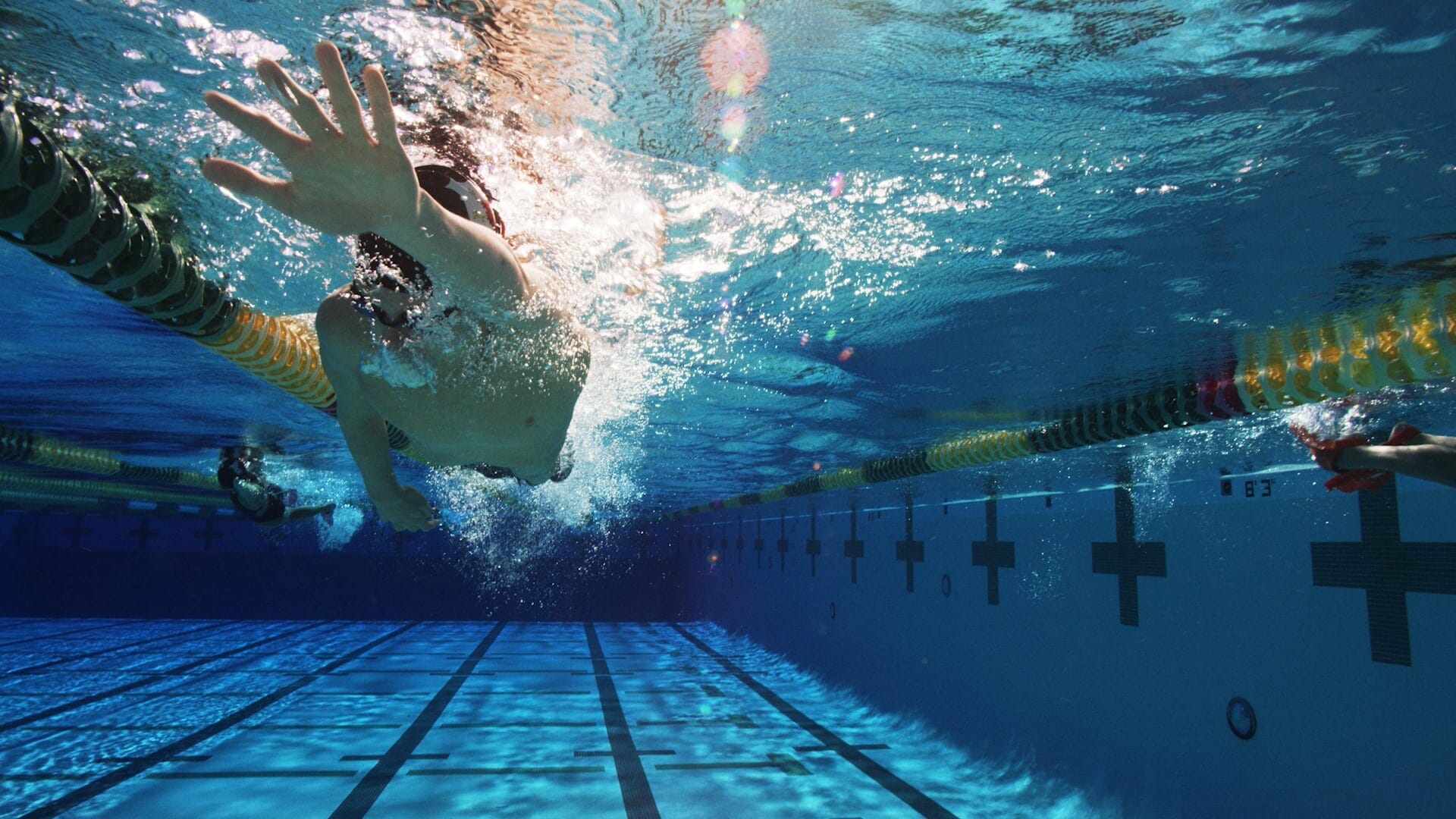This underwater photograph vividly captures the dynamic scene of a swimming competition. In the turquoise, sparkling waters of the pool, highlighted by bright, cheerful hues, two shirtless male swimmers are seen in action. Their powerful strokes create an explosion of bubbling white foam at the surface. The primary swimmer, positioned centrally and slightly to the left, stretches one hand forward while the other trails behind, displaying a determined pace. He appears to have shorter, dark hair and is adorned with a swim cap. The second swimmer is visible in the background on the left, diving into the pool with forceful energy. Sunlight streams down from above, illuminating the scene and casting a vibrant light blue hue across the water. Distinct dark black crosses adorn the pool walls, and lane markings delineate the swimming lanes, emphasizing the competitive nature of the moment.